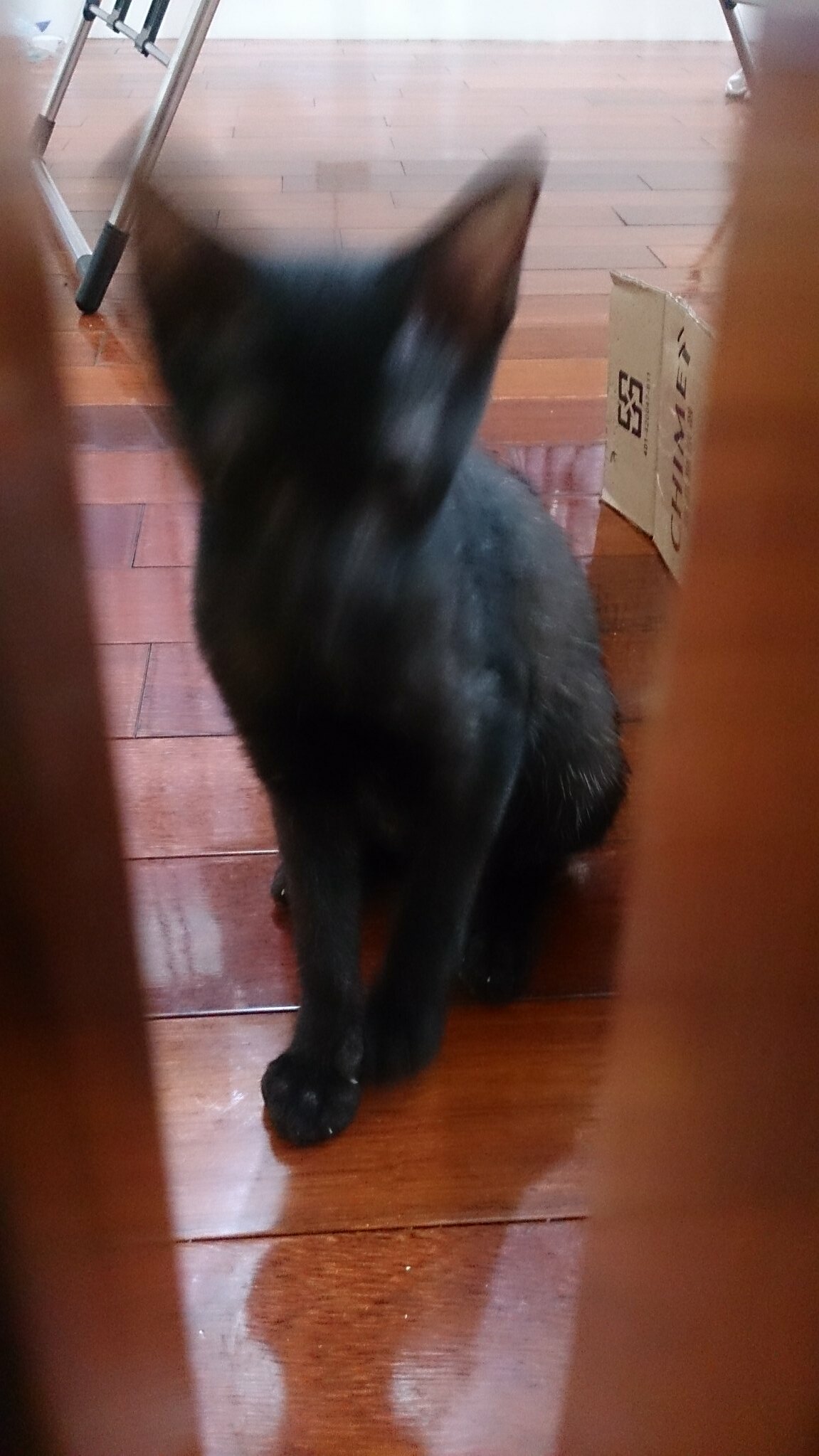A vertical image captures a dynamic scene with noticeable motion blur, suggesting the subject's swift movement. A black cat sits on a glossy, mahogany-brown wooden floor, its tall ears standing out sharply against the blurred surroundings. The cat's head is in motion, resulting in a blurred face that conveys a sense of activity and restlessness. The sides of the image are partly obscured by similar brown-colored elements, likely wooden slats from a fence or railing, creating a framed view of the scene as if peering through a small window.